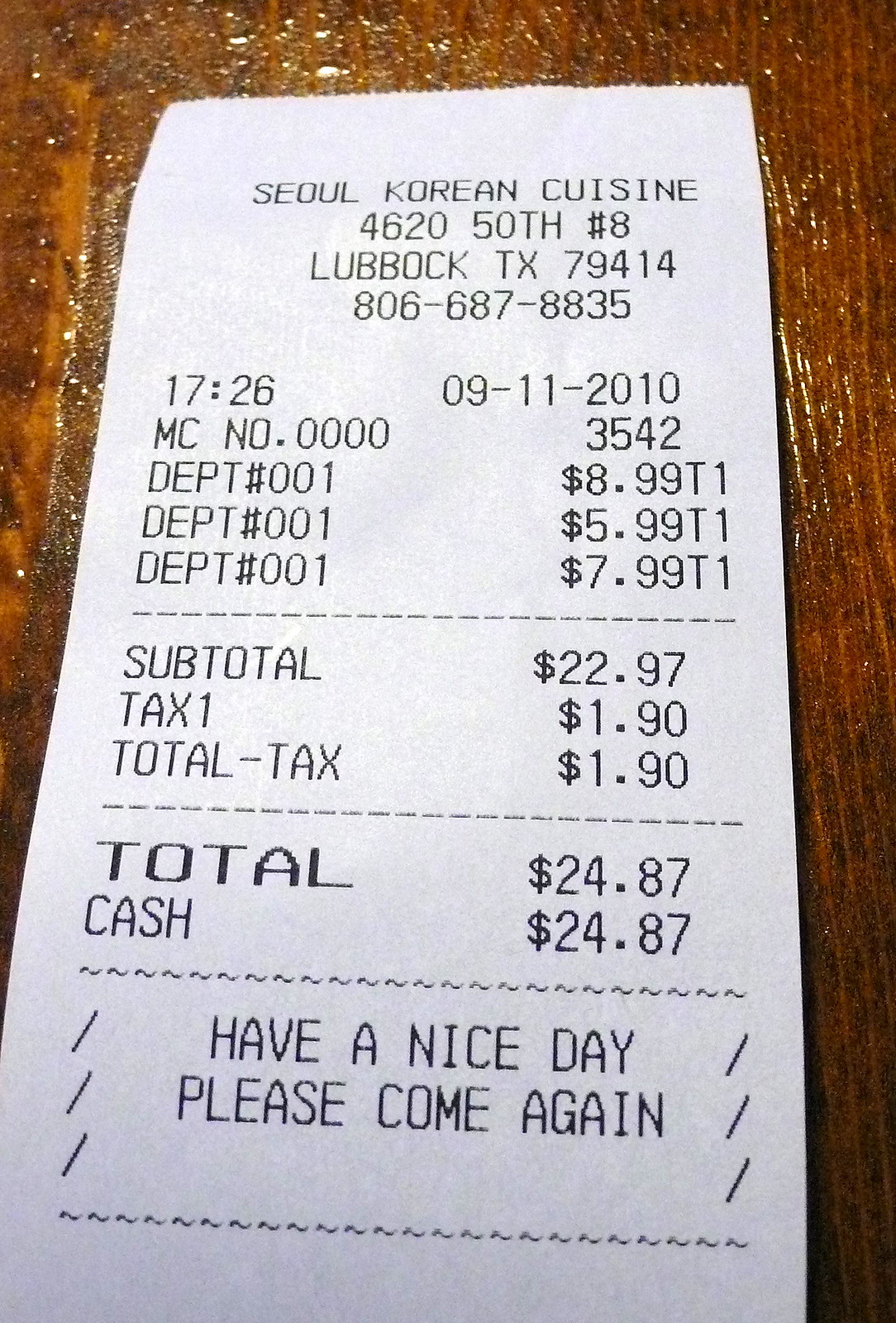A receipt from Seoul Korean Cuisine is placed on a wooden table. The restaurant’s address, 4620 50th St, Unit 8, Lubbock, Texas, 79414, and phone number, 806-687-8835, are printed beneath its name. The transaction took place at 17:26 hours on September 11th, 2010. The receipt includes a merchant code "MC NO. 0000" and a reference number "3542" on the right side.

In the itemized section, three departments are listed:
- Department No. 001: $8.99
- Department No. 001: $5.99
- Department No. 001: $7.99

The subtotal amounts to $22.97, with a tax of $1.90, bringing the total to $24.87. The payment was made in cash. At the bottom, a friendly message reads, "Have a nice day, please come again."